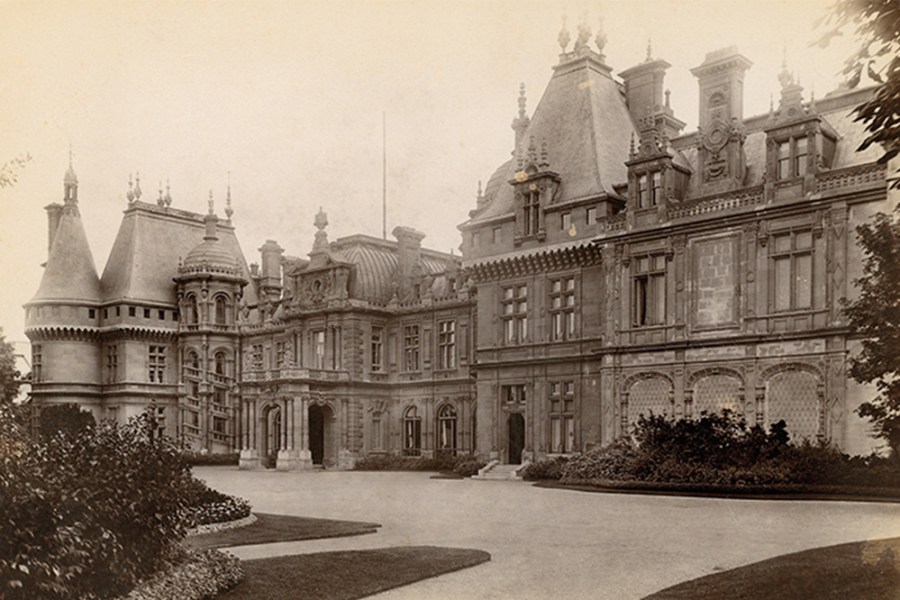This image is an old, horizontally oriented photograph of a grand mansion or castle, likely taken during the day. The photograph has aged significantly, displaying a yellowed and faded sepia tint, indicative of its age, possibly around 100 years old. The mansion, potentially Victorian in style, is depicted with high, pointy roofs and intricate architectural details including decorative carvings, trims, and moldings. The building consists of multiple elaborate windows and stone walls, suggesting just one wing of a presumably larger structure, spanning perhaps 100 to 200 feet wide. 

In the foreground, there is a driveway leading up to the mansion, flanked by grass, shrubs, trees, and flowers visible on the bottom left and right of the image. The landscape around the mansion includes bushes and other landscaping elements. The image also captures various structural details like steeples and a brick wall between some windows on the right-hand side, as well as steps leading to the front door in the center of the scene. The overall ambiance of the photograph speaks to a grand and opulent era, with a lightly clouded sky providing a backdrop to the aged elegance of the mansion.